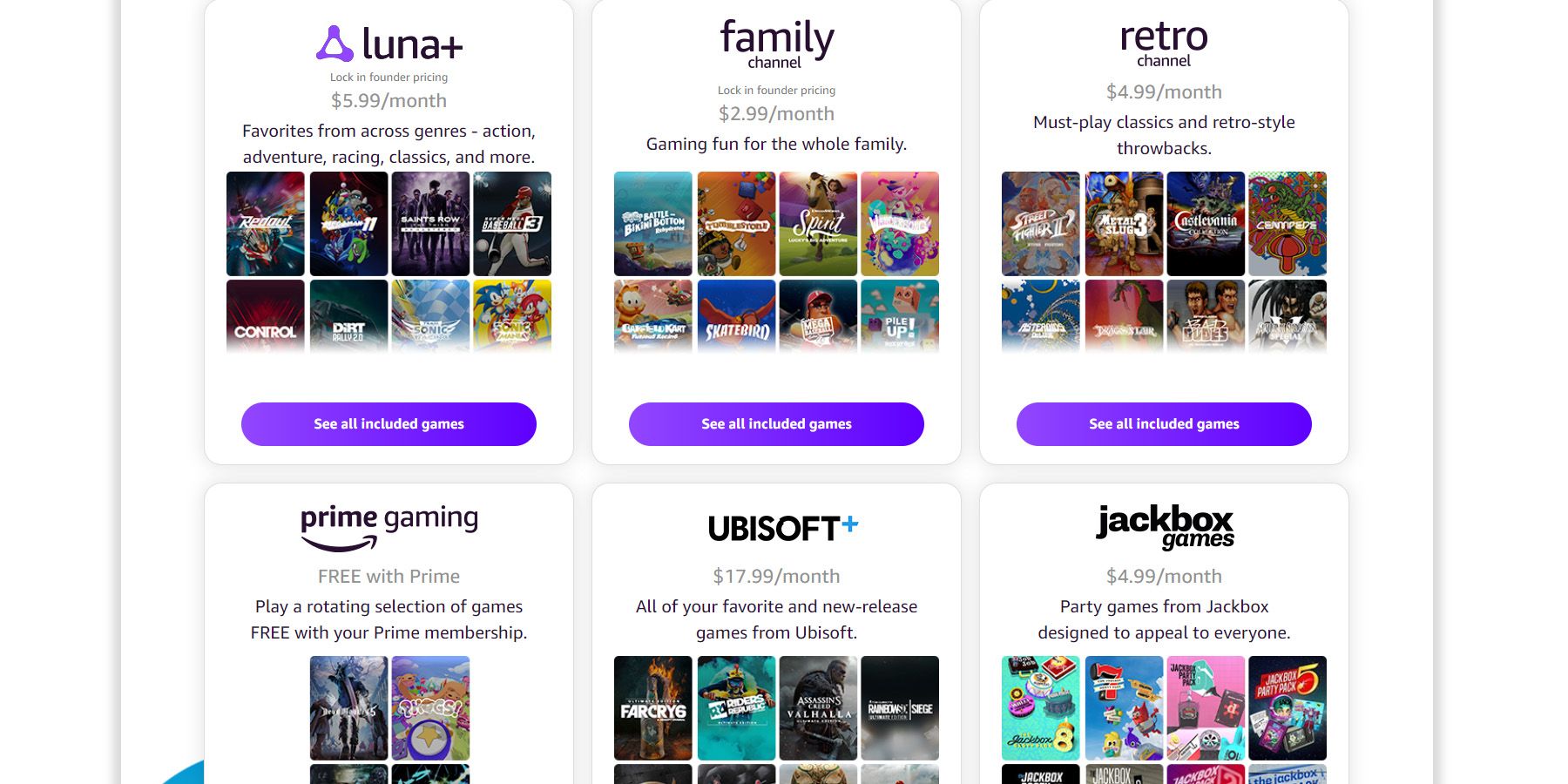This promotional image showcases various gaming subscription options available through Amazon Luna. At the top of the image, the Luna Plus plan is highlighted in bold, offering a diverse library of action, adventure, racing, and classic games for $5.99 a month. Directly to the right, the Family Channel is featured, costing $2.99 a month and offering gaming experiences suitable for all family members. Adjacent to it, the Retro Channel is detailed, priced at $4.99 a month and focusing on must-play classics and retro-style throwbacks. 

Beneath these options, an emphasis on "Gaming Free with Prime" is made, allowing Prime members to enjoy a rotating selection of games at no additional cost. Beside this, the Ubisoft channel is promoted for $17.99 a month, granting access to popular and newly released Ubisoft titles. Lastly, the Jackbox Games channel is presented at $4.99 a month, offering a range of party games designed to entertain all audiences.

A prominent purple and white button at the bottom of the image invites viewers to "See All Included Games," encouraging further exploration of the gaming selections available.